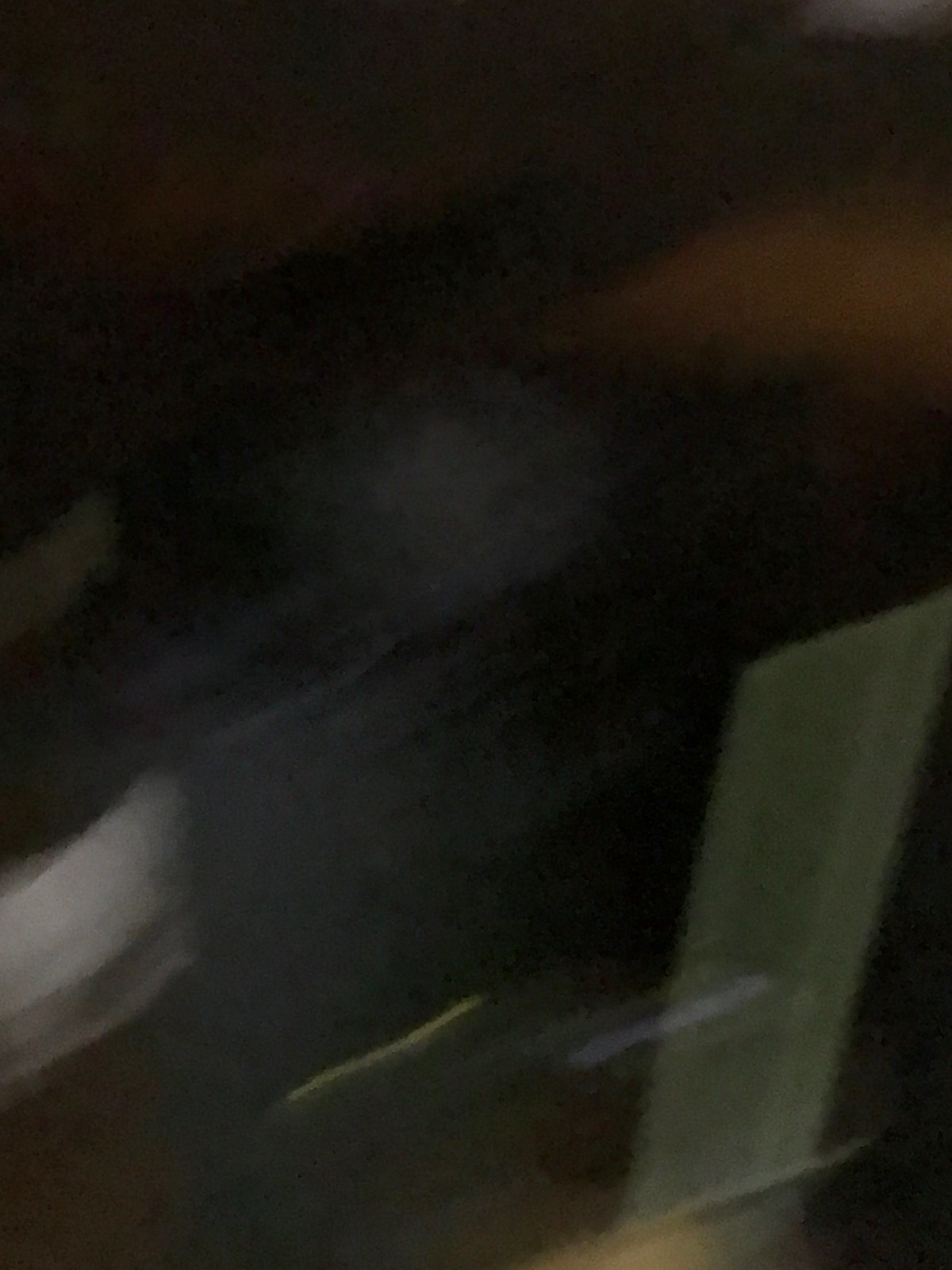An extremely blurred image captured at night, likely from within a moving vehicle such as a car or bus, showcases a complex interplay of lights and motion. The left half of the image is predominantly black, extending diagonally from the top right corner to just below the center on the left side, suggestive of a dark interior space. In the bottom right section, a white rectangle, possibly a light source or a door, creates a stark contrast amidst the surrounding darkness. This area also features elongated light trails caused by the camera's movement during the shot. 

Near the lower left corner, a white section suggests the presence of a sleeve, while adjacent to it, a hazy blue area hints at an article of clothing, perhaps a jacket or waistcoat. Adding to the color spectrum, the top right corner of the image displays an indistinct orange blur, providing a touch of warmth to the otherwise cool-toned and shadowy scene. The overall effect is a chaotic yet intriguing blend of motion, light, and darkness, capturing a fleeting moment enveloped in nocturnal mystery.